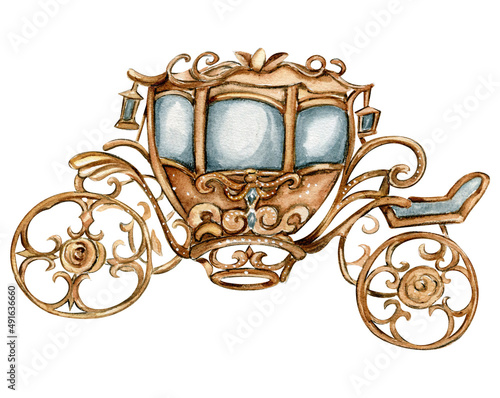The image features a detailed, watercolor or marker illustration of an ornate, upper-class horse-drawn carriage, reminiscent of Cinderella's fairy-tale transport, set against a white background. The carriage, primarily light brown or brass in color, is adorned with intricate wooden shapes and designs. Prominent blue-tinted windows and a matching blue seat enhance the carriage's elegance, with turquoise and white jewels adding a touch of sparkle. Two brass lanterns with turquoise windows are positioned at the top left and right corners, contributing to the carriage's luxurious appearance. The two large wheels are notable for their intricate curlicue patterns, both within the spokes and along the outer edges. In the lower left-hand corner of the image, the text "Adobe stock number 491636660" is printed vertically in small type.